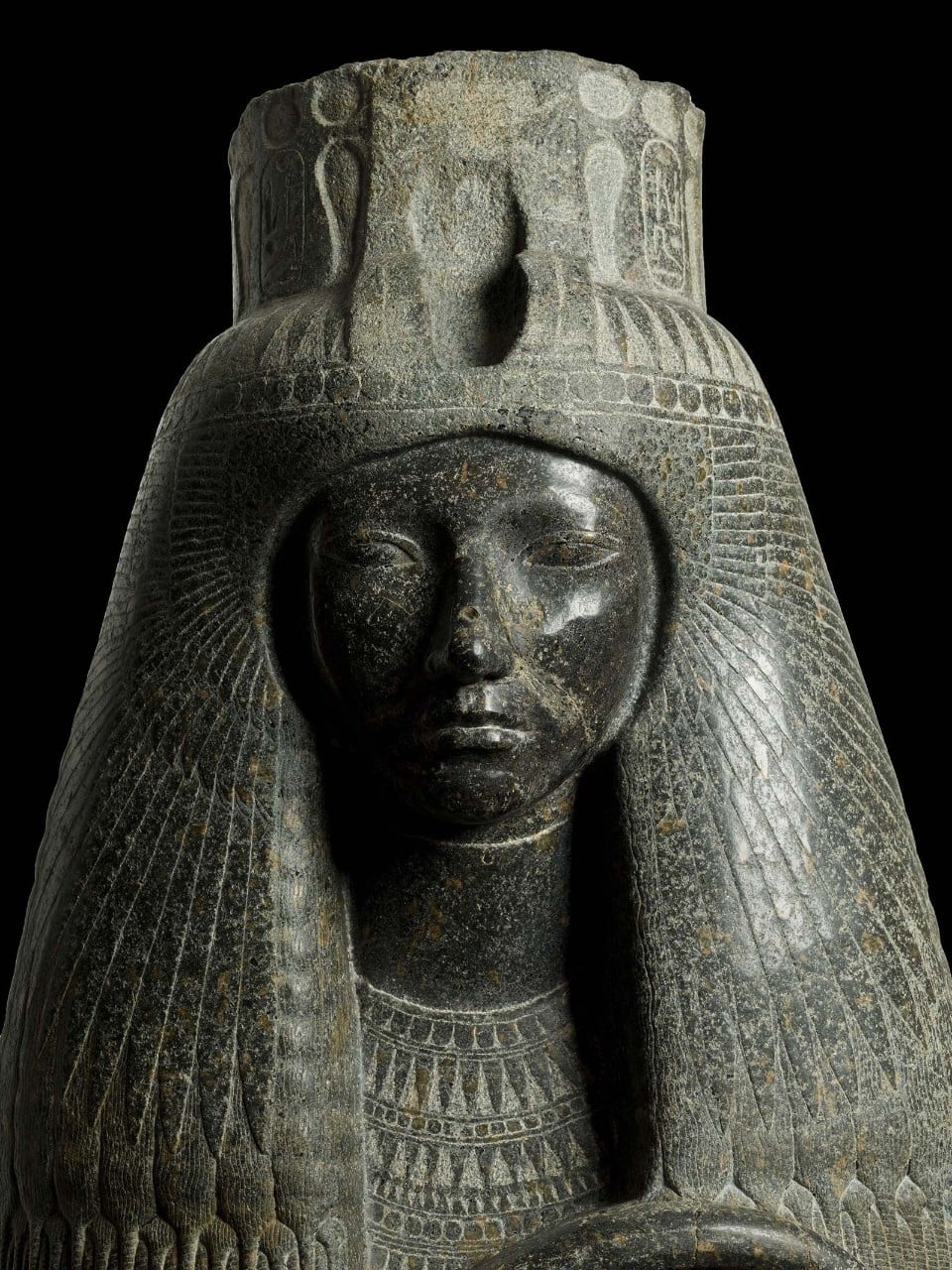This image showcases a close-up photograph of a finely crafted statue against a dark black background. Carved from smooth, dark gray stone—possibly granite or marble—the statue depicts a regal female figure evocative of Egyptian or African heritage. Her eyes are closed, with well-defined eyebrows, a broad nose, and a serious, unsmiling expression on her lips. She is adorned with an elaborate headdress and an ornate necklace. 

The headdress is particularly striking, featuring a cylindrical top that extends 6 to 8 inches above her head, decorated with symmetrical circular patterns. This crown-like structure appears slightly worn at the top, with a central vertical groove suggesting the prior presence of a jewel or ornamental piece. The headdress also includes intricate feathered patterns and a band of circular motifs just above her eyes, enhancing her regal appearance.

Around her neck, an ornate collar extends down over her chest, adding to the statue’s majestic aura. The statue is elegantly lit from the right, emphasizing its intricate details against the deep black background, making it a likely fixture in a tomb or a traditional celebratory context.